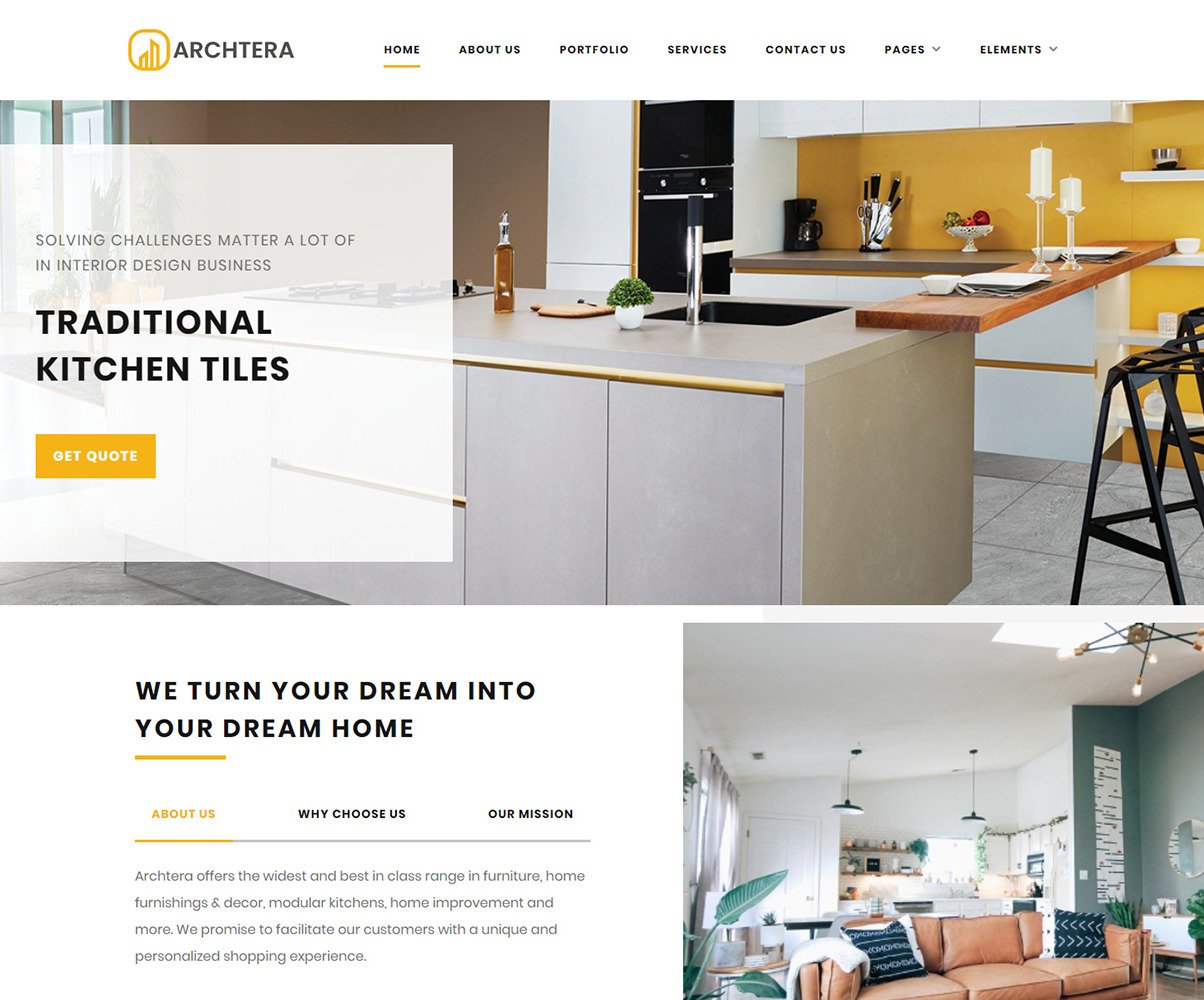Screenshot of the Architera website: 

The website, named "Architera" (spelled A-R-C-H-I-T-E-R-A), features a distinctive logo of two stylized yellow buildings. The site's navigation menu, displayed horizontally from left to right, includes the following options: Home, About Us, Performative Services, Contact Us, Pages (with a pull-down menu), and Elements (with a pull-down menu). The 'Home' tab is currently selected and highlighted with an underlined yellow bar.

The main content section showcases an image of a modern kitchen. The kitchen features white cabinets, a fold-down countertop (now discontinued due to safety concerns), kitchen knives in a block, and a built-in wall oven. The sink is centrally placed, an unusual choice. Overlaying this image is a semi-transparent white box with the text, "Solving challenges matter." 

Below this, an additional text banner reads, "We turn your dream into your dream home," with 'your' emphasized by yellow underlining. Further descriptive text in yellow shares, "Architera offers the widest and best-in-class range of furniture, home furnishings, decor, modular kitchens, home improvement, and more. We promise to facilitate our customers with a unique and personalized shopping experience." 

To the right of this text, black headings read, "Why Choose Us" and "Our Mission." Adjacent to the text is an image showing a cozy couch, with what appears to be a small kitchen area in the background, reinforcing the theme of home renovation and interior design. 

Overall, the layout and imagery convey Architera's dedication to quality and personalized home improvement solutions.